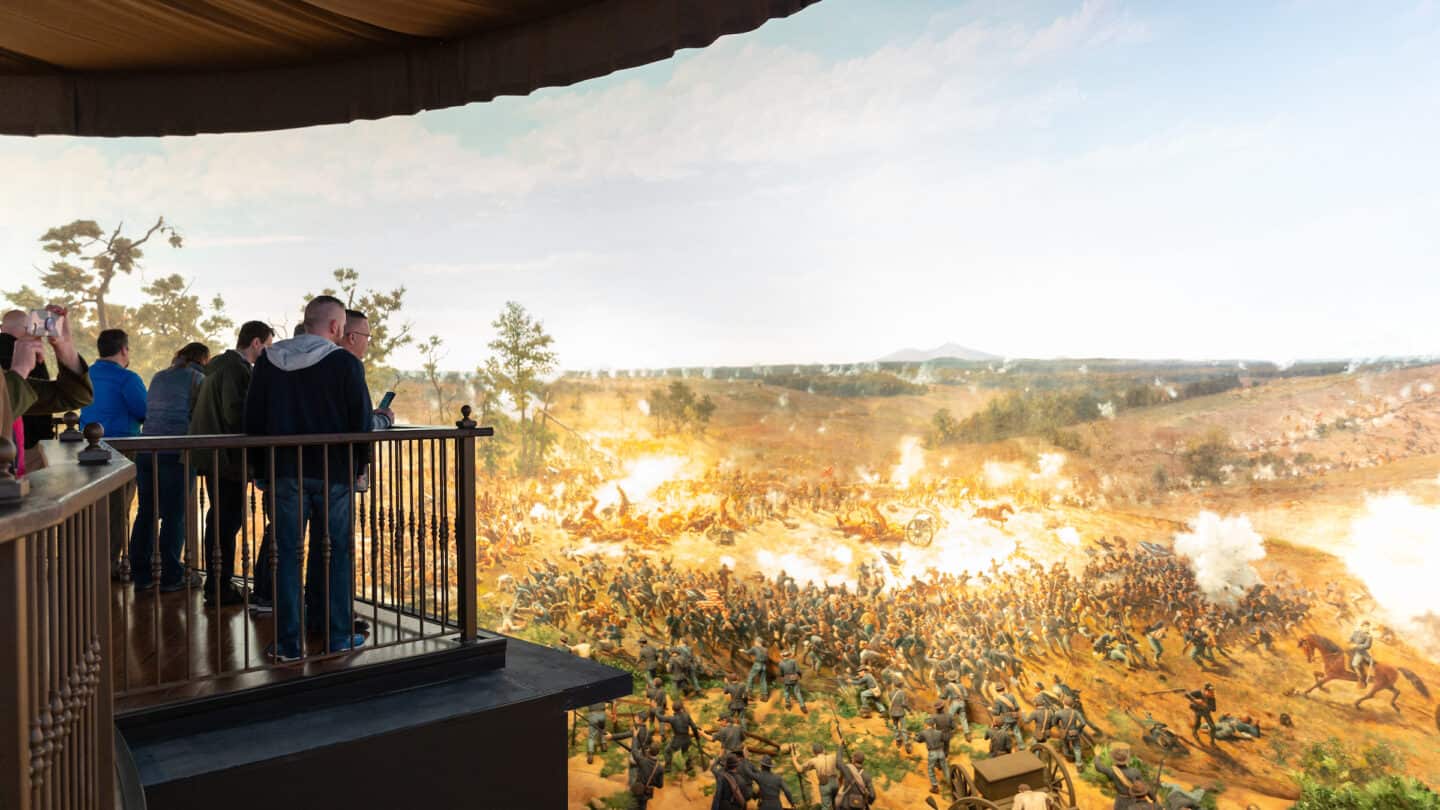The image captures a group of people standing on a curved, black-painted wooden balcony with a brown metal railing in the top left corner. They are observing what appears to be an ornate display on a large wraparound screen that seamlessly blends photographic and illustrative elements. The individuals, some taking pictures with their phones, are situated in an indoor environment suggested by the visible curtains draping around the scene. The display on the screen vividly depicts a chaotic battle on an open dirt plain, where soldiers, some mounted on horses, are engaged in combat amidst smoke, fire, and explosions, evoking imagery reminiscent of the Civil War. The background showcases elements like a blue sky with clouds, distant mountains, and scorched trees, enhancing the immersive and dramatic nature of the scene.